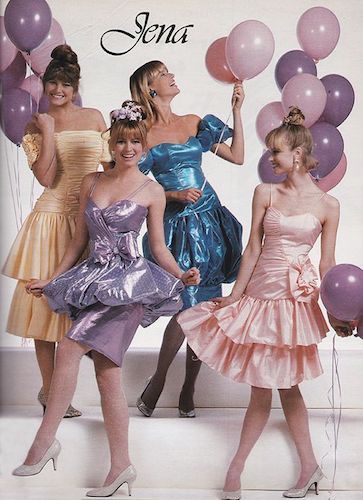The image appears to be a vibrant catalog or magazine photo from the late 80s, featuring four women in party dresses, likely in their late 20s to early 30s. They are captured standing on various steps, adding a dynamic staggered effect. The woman on the far left is poised with her arm raised, flaunting an off-the-shoulder yellow dress adorned with two flounces. Beside her, a lively woman is lifting her leg, showcasing a striking shiny purple dress with straps and a large bow. Next to her is a woman in a dazzling metallic teal dress with puffed sleeves and black stockings, radiating a blend of elegance and fun. The woman on the right rounds out the group with a light pink dress featuring two flounces and straps. Surrounding the women are bunches of pink and purple balloons, heightening the festive atmosphere. Above the scene, in bold black script, the text "Jena" is spelled out, adding a touch of branded sophistication to the lively ensemble.